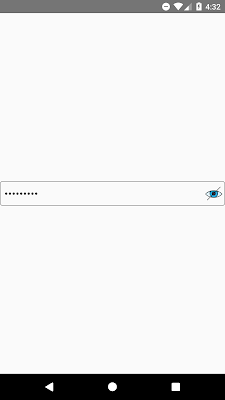The image is a screenshot displaying a password entry interface. At the top of the screen, there's a thin gray rectangle containing a white circle with a gray minus sign, icons indicating full Wi-Fi signal and half cellular service, and an upright battery icon with a lightning bolt, suggesting it's charging. The image is somewhat pixelated, and the time captured is 4:32. The website's purpose isn't specified; central to the image is a password field represented by a horizontal rectangle filled with nine small dots, denoting the concealed characters. To the rectangle’s far right is an eye icon with a slash through it, indicating the password is hidden. At the bottom of the screenshot, navigational buttons include a back arrow on the left, a circle in the center, and a square icon resembling a pause button on the right.